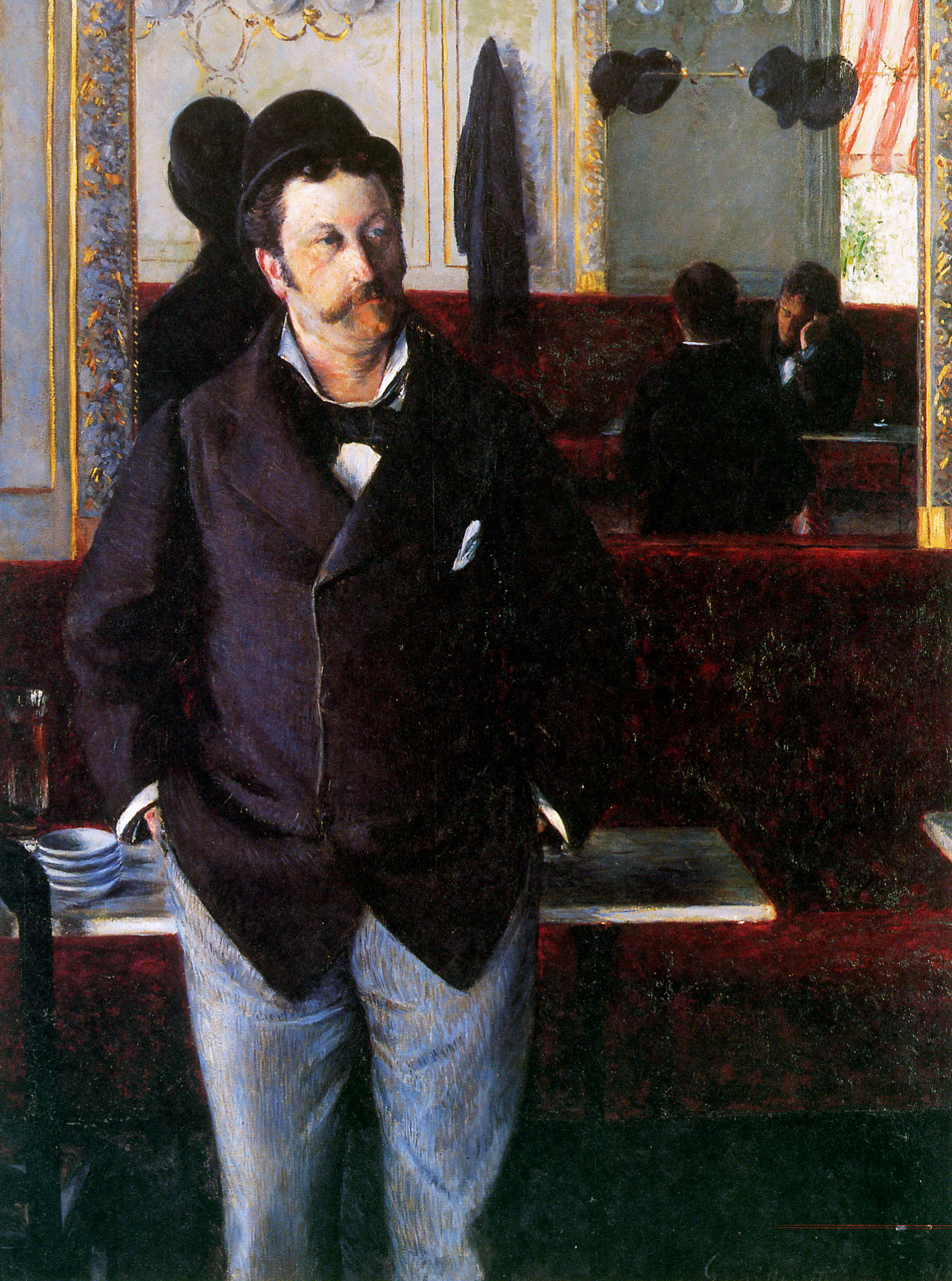This detailed painting depicts a contemplative man standing indoors, dressed in a black buttoned jacket adorned with black buttons, a white collared shirt, and a black bow tie. He is also wearing a black bowler hat, with well-groomed sideburns and a long mustache on his roundish face. Positioned from about the knees up, the man stands in front of a large mirror, which reflects the back of his head and hat, as well as some elements of the background.

Behind him, the mirror reveals a scene of a lavishly decorated restaurant, adorned with rich gold fillory accents. In the background, two men are seated at a table covered in dark red velvet. One man is leaning his head against his hand with his elbow on the table, while the other, seen from the back, also wears a black jacket. There are additional details like a striped red and white awning visible through a window, hats and a jacket hanging on bars protruding from the wall, and a table countertop below him with bowls and dishes. The color palette of the painting includes black, white, gray, red, maroon, yellow, gold, peach, orange, blue, and silver, combining to create a slightly abstract yet recognizable scene.